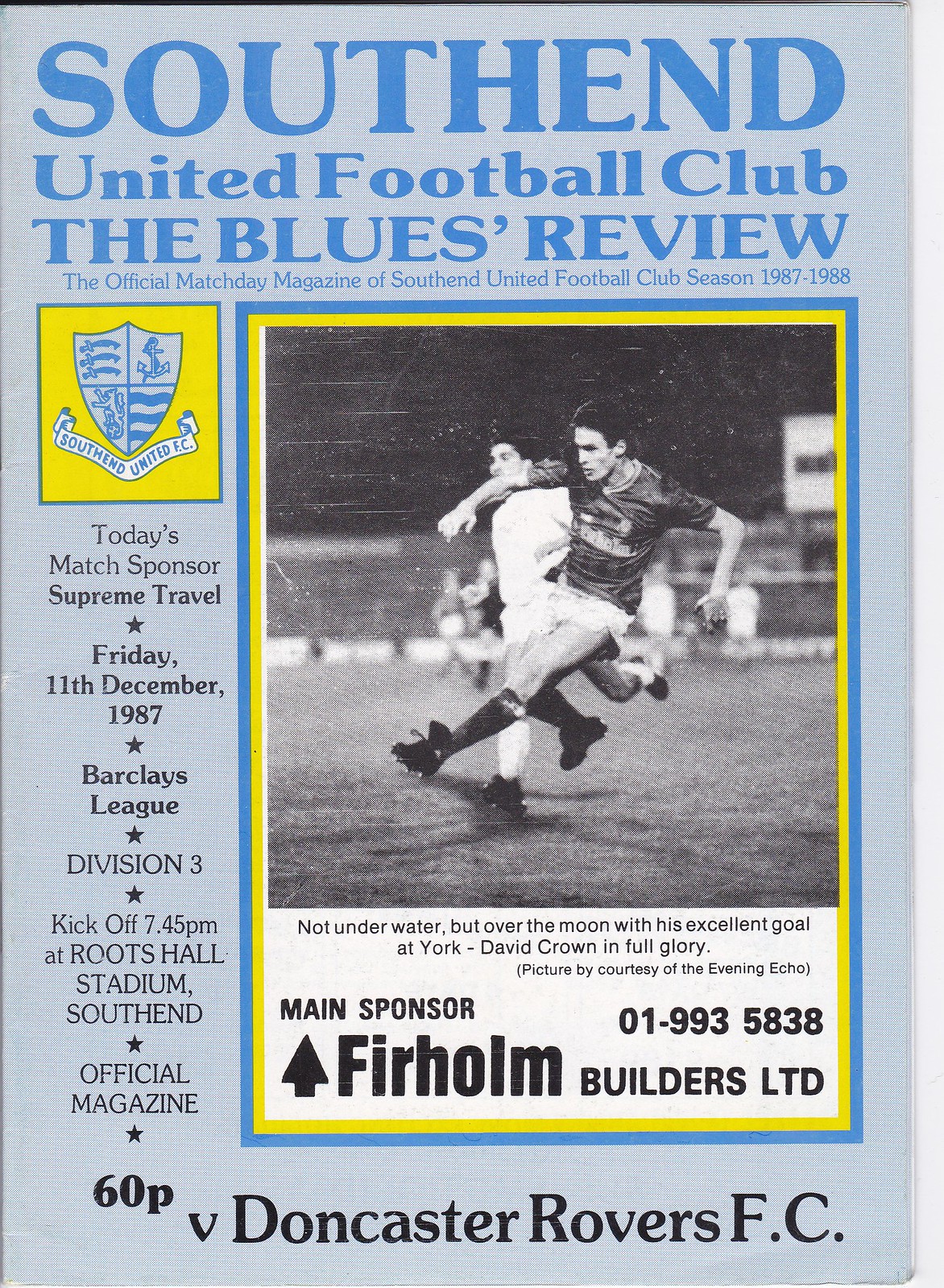This vintage cover of the South End United Football Club's official matchday magazine, "The Blues Review," from the 1987-1988 season, is designed with a light blue and white background, enhanced by a rectangular layout that is taller than it is wide. The top of the cover features the title "South End United Football Club, The Blues Review" in bold blue letters. Beneath it, the small print describes the magazine as "the official matchday magazine of South End Football Club season 1987-1988."

On the left side of the cover, there is a small yellow rectangle with a blue outline, containing a blue and white crest. The crest is divided into four quarters: three swords in the upper left, an anchor in the upper right, a rearing lion in the lower left, and three blue wavy lines in the lower right. Below the crest, a banner reads "South End United." Additionally, the text along the page's left side lists details about the match: "Today's Match Sponsor, Supreme Travel," "Friday, 11th December 1987," "Barclays League Division III," "Kickoff 7:45 PM at Roots Hall Stadium, South End," and "Official Magazine, 60p."

The bottom of the cover features "V. Doncaster Rovers FC." The right portion of the cover is dominated by a framed black-and-white photograph of two soccer players in action, outlined by a blue pinstripe and then a yellow border. The text underneath the photo reads, "Not underwater but over the moon with his excellent goal at York, David Crown in full glory," with credit to "The Evening Echo." At the very bottom, it notes "Main Sponsor: Firholm Builders Ltd, 01-993-5838."

This detailed magazine cover exudes a nostalgic charm from the late 80s, capturing the essence of a classic football club advertisement.